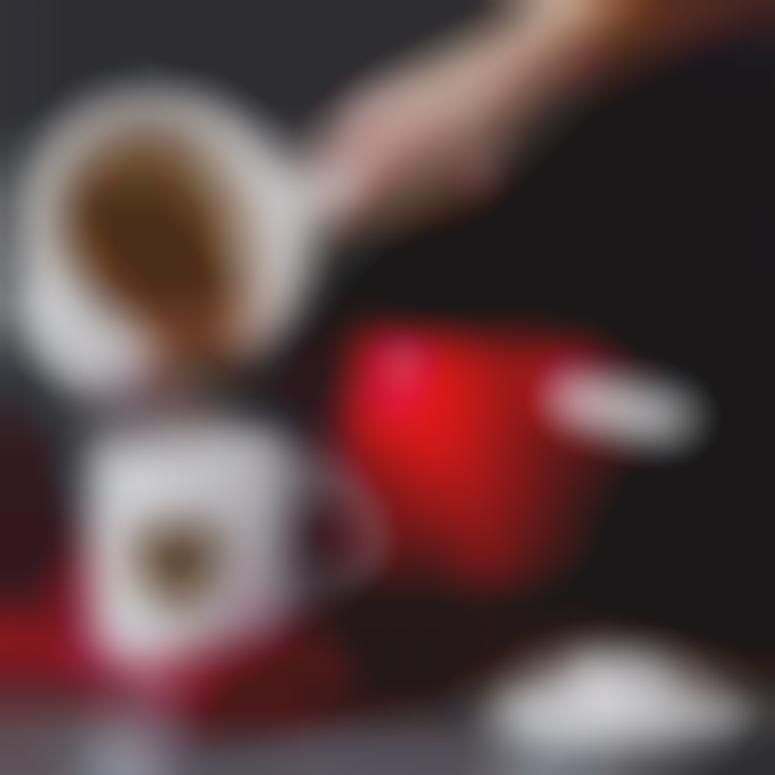The image is a large, rectangular, and notably blurry photograph that captures what seems to be a hand pouring a brown liquid—presumably coffee—from a larger white mug or pouring dispenser into a smaller white cup below it. The smaller cup appears to have a brown dot or logo on it. To the right of this scene, there is a larger red pot with a white handle. The background is predominantly black, with a black surface on which some objects rest. Due to the severe blurriness of the photograph, the details are difficult to discern, necessitating some assumptions about the contents and context.